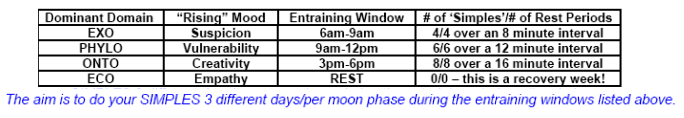This image is a detailed text infographic styled in black and white, with four columns and five rows, including the header row. The table is arranged horizontally, and each column is outlined in black.

The headers of the columns are, from left to right: "Dominant Domain," "Rising Mood," "In Training Window," and "# of Symbols/# of Rest Periods." 

The first column lists EXO, PHYLO, ONTO, and ECO. The second column associates these with moods: suspicion, vulnerability, creativity, and empathy, respectively. The third column provides timeframes: 6 a.m. to 9 a.m., 9 a.m. to 12 p.m., 3 p.m. to 6 p.m., and REST. The fourth column indicates symbols and rest intervals: 4/4 over an 8-minute interval, 6/6 over a 12-minute interval, 8/8 over a 16-minute interval, and 0/0 noted as a recovery week.

Under the chart, written in blue text, is a footnote that reads: "The aim is to do your samples three different days per moon phase during the in training windows listed above."